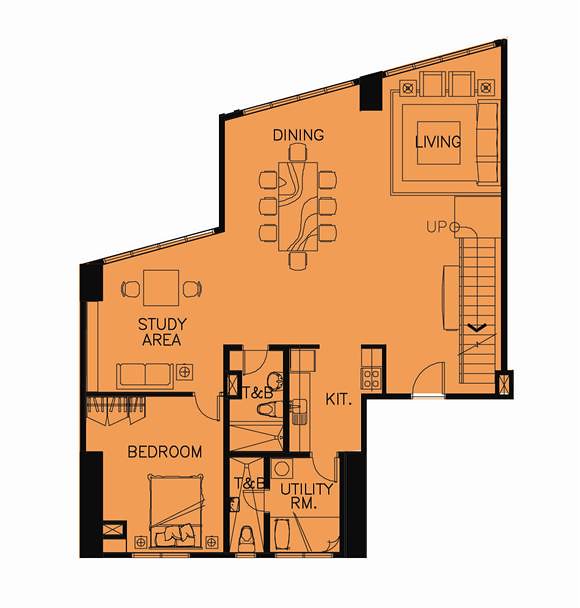Detailed Caption:

The image depicts a detailed floor plan of a building, divided into various clearly labeled areas. At the top, there's a dining area featuring a rectangular table surrounded by chairs. Adjacent to the dining area, on the top right, is the living room, furnished with a couch on the right side and two additional seats at the top. In the middle of the layout are several squares, possibly representing additional furniture or utility spaces. The far-right section is labeled "You Peel," accompanied by an arrow pointing downward, indicating the presence of stairs.

On the bottom side of the plan, there's a door depicted as swinging open, leading outside. Moving leftward from the door is the kitchen, complete with a stove and a sink on the left side. Further left, the plan reveals a utility room containing various utilities. Adjacent to the utility room is a space labeled "T&B," which likely stands for toilet and bath; it includes a toilet at the bottom and a sink.

To the left of the kitchen, there’s another "T&B" area, featuring a sink, a toilet, and additional unspecified fixtures at the top. Further left, a study area is displayed, equipped with a table, two desks or chairs, a couch, and a side table with a lamp. Finally, the bottom left section houses a bedroom with a bed in the center, flanked by furniture on both sides and neighboring a closet with hangers. The perimeter of the floor plan is bordered, and window locations are indicated by rectangular shapes with bars through them.